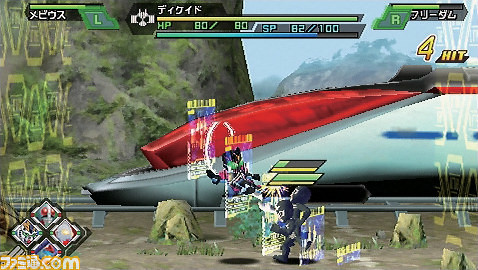In this image, we see a screenshot from an Xbox video game, indicated by the logo in the upper left corner. The top part of the screen features a snippet of Chinese text, highlighted by a blue underline with a yellow background. To the right, there are numerical stats displayed: "80/80" and "SP82/100". Additionally, a green square with a letter "R" inside is also visible. The text "Four Hit" appears prominently in bold yellow letters.

At the center of the screenshot, there is a striking depiction of a white jet with blue-tinted windows and a distinctive red stripe running along its front. The lower portion of the screen contains various icons and game-related information, likely representing scores and other in-game statistics.